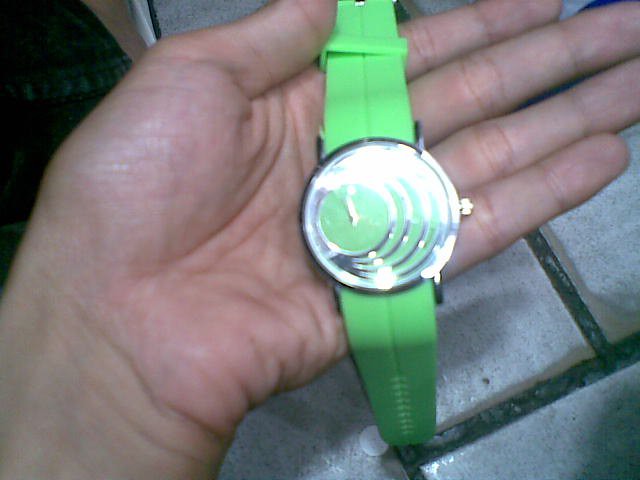This somewhat blurry, up-close photograph features a left hand holding, not wearing, a neon green-banded watch with a unique face design. The wrist and the fingers, specifically the middle and ring fingers, are partially visible, with the fingers extending out of the upper right corner of the frame. The neon green wristband offers a stark contrast to the background, which consists of square gray tiles with dark gray grout. The watch face is characterized by concentric circles of silver and green, with the innermost circle housing two hands that suggest the time is near noon or midnight. Due to the glare on the watch face, finer details are obscured, making the design challenging to discern. There appears to be a hint of additional background elements, possibly including a piece of a cabinet.